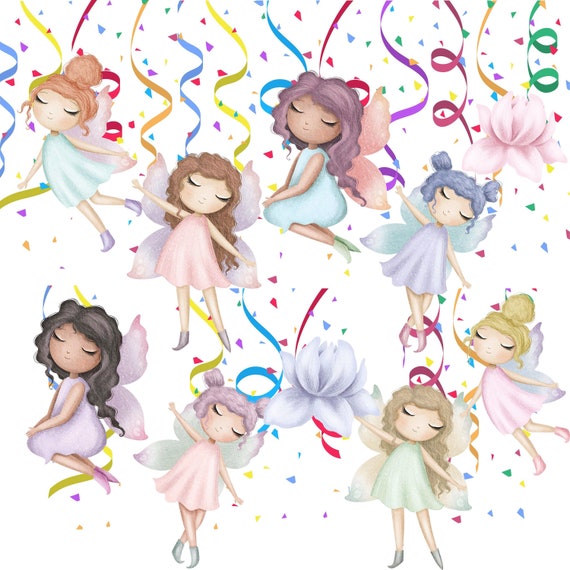This illustration features eight whimsical cartoon fairies arranged in two rows of four. Each fairy has a distinctive appearance with big heads, large eyes, and small mouths, giving them a charming, childlike look. Their eyes are closed, accentuated by long, upward-swooping lashes, and smiles grace their faces. The fairies have varied hairstyles, including long hair, short hair, buns, and space buns, in different colors. They wear simple, identical dresses in vibrant pastel shades of purple, pink, blue, and green, complemented by matching wings.

The background is a festive sea of birthday confetti, streamers, and ribbons, creating a playful contrast with the fairies. Two flowers are nestled among the fairies - one above the top right fairy and another between the two fairies on the bottom row. Some fairies are depicted standing, while others appear to be floating or posing, adding dynamic movement to the scene. The overall effect is a delightful, colorful celebration of these enchanting fairy characters.